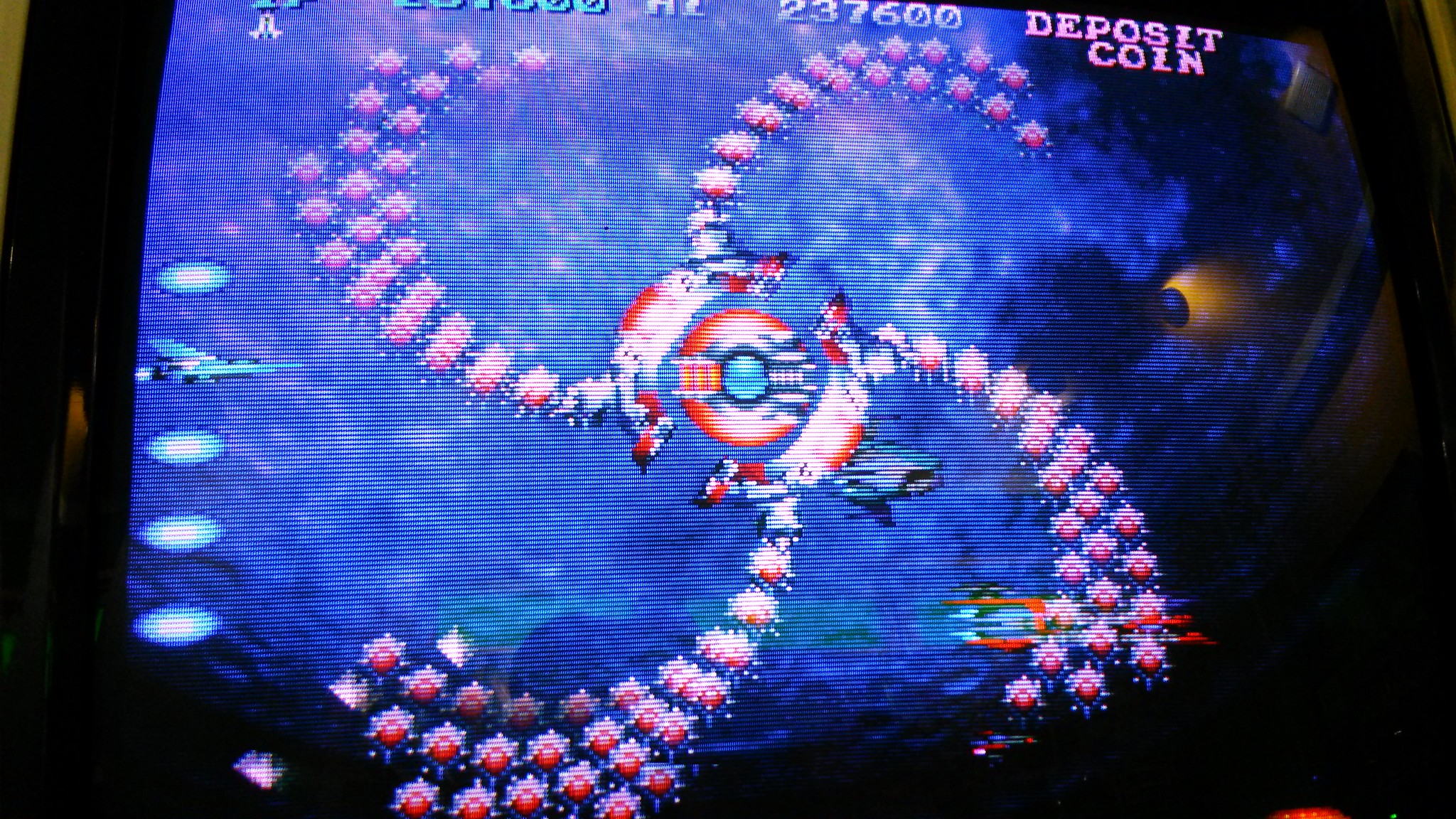This image captures a TV screen displaying an underwater-themed video game in progress. The primary focus is on the top right corner, which prompts "Deposit Coin." Just to the left is the score, proudly showcasing a high score of 237,600 points. Further to the left, additional numerical data can be partially seen, though not clearly enough to discern. The in-game action reveals a dynamic scene with characters moving in a circular pattern, exuding visual effects such as stars, which are later identified as bombs. Among the elements in the game environment are a prominently featured shark, several floating pressure mines, and an array of bubbles, contributing to the immersive underwater experience.